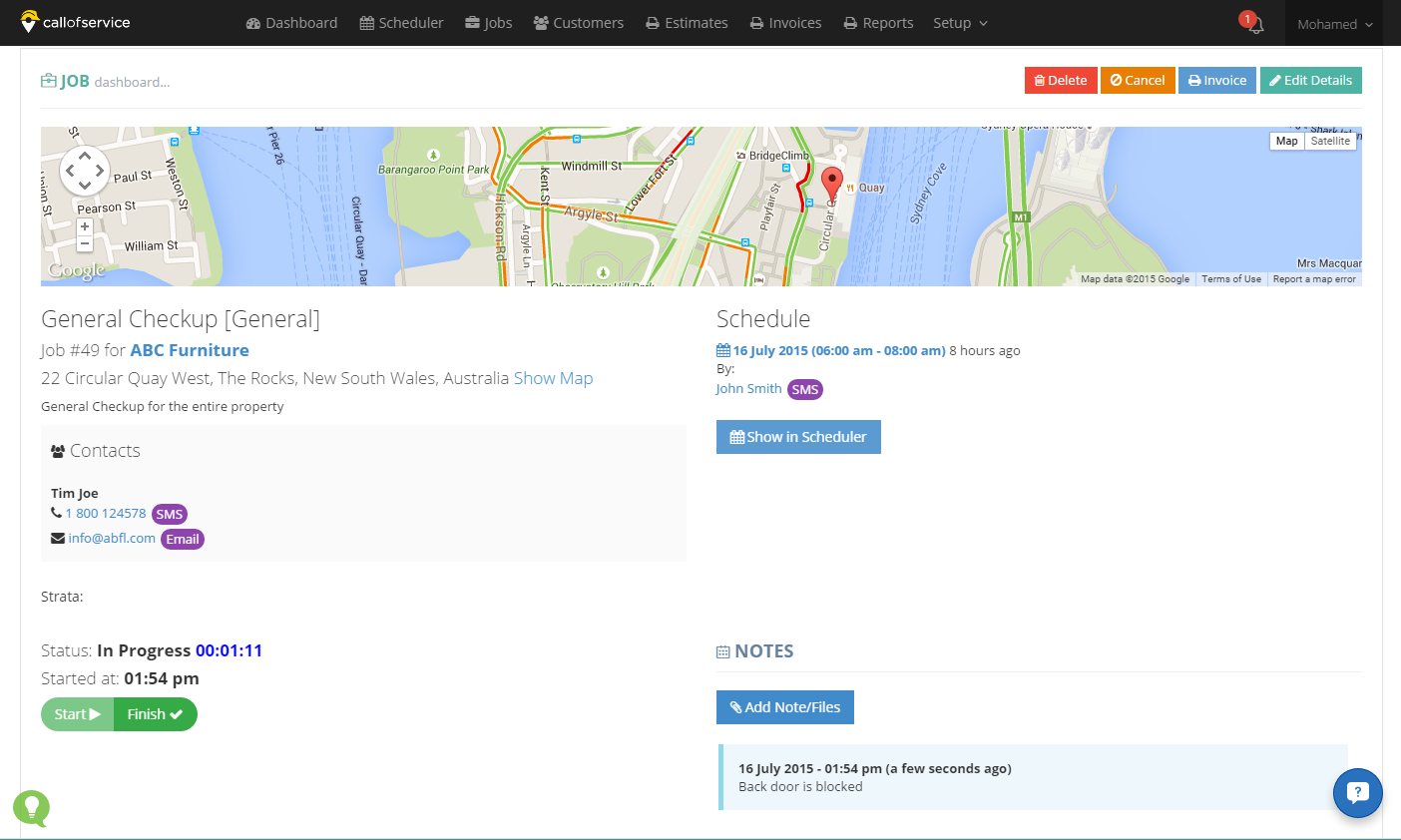The image depicts a detailed map with a variety of overlays and informational elements. The top portion of the map is set against a solid white background and features a long black triangular section. This section includes a navigation menu with white text, though the text is somewhat small and difficult to decipher. The menu options appear to include "Dashboard," "Schedule," "Jobs," "Documents," "Projects," "Reports," and "Setup," the latter accompanied by a downward-pointing arrow.

Below this menu, within the white box, the map interface begins. At the top of this section, there is a label marked "Job" with several buttons to the right, such as "Invoice," "Edit Details," and other action items. The map itself displays a location named "General Checkup (General)" for ABC Furniture located in Australia. The map highlights various geographical features including bodies of water and green areas, with a notable red mark on the left side of the map.

Underneath the map, there is a "Contacts" section listing a phone number, accompanied by the "Status and Progress" indicator showing a timestamp of 1 minute, 11 seconds, suggesting an ongoing call that started at 1:54 PM. 

On the right side, below the map, there is a "Schedule" section indicating a date of July 18th, 2015, along with options to show schedule events or settings. Finally, at the bottom of the image, there is a menu for "Notes" with an option to add new notes.